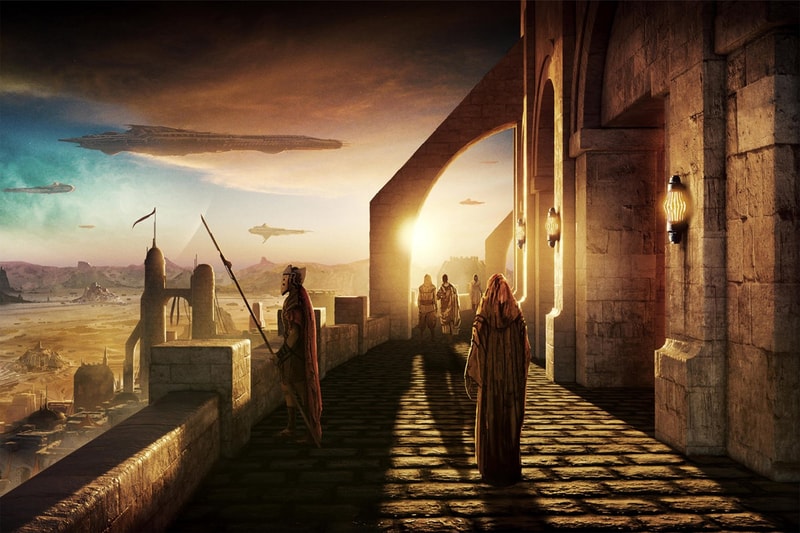The image appears to be an intricate and colorful artistic drawing that depicts a fusion of medieval and futuristic elements set in a kingdom high above the ground. To the center and right, a figure in long robes walks along a parapet or sidewalk, heading towards the viewer. To the left, a soldier in medieval attire, holding a spear, stands guard, gazing outward. The parapet runs along the side of a large castle or fortress with stone tiles and walls, exuding a medieval ambiance while being part of a high-tech world.

In the background, we see buildings that suggest another castle-like structure, reinforcing the medieval aesthetic. However, the futuristic aspect is highlighted by various flying devices—spaceships, drones, helicopters, and small airplanes—traversing the sky. The sky itself dazzles with vibrant hues of beige, light blue, purple, and white, adding to the otherworldly atmosphere. The sun shines brightly, illuminating the scene with an almost ethereal glow.

Additional details include distant mountains and possibly sandcastle-like formations to the left, as well as flags hanging from structures and lamps near arched doorways that adorn the castle. This surreal scene is set against a backdrop of a sky filled with violet-tinged clouds and patches of blue, capturing the essence of an advanced civilization seamlessly blending medieval and futuristic elements.